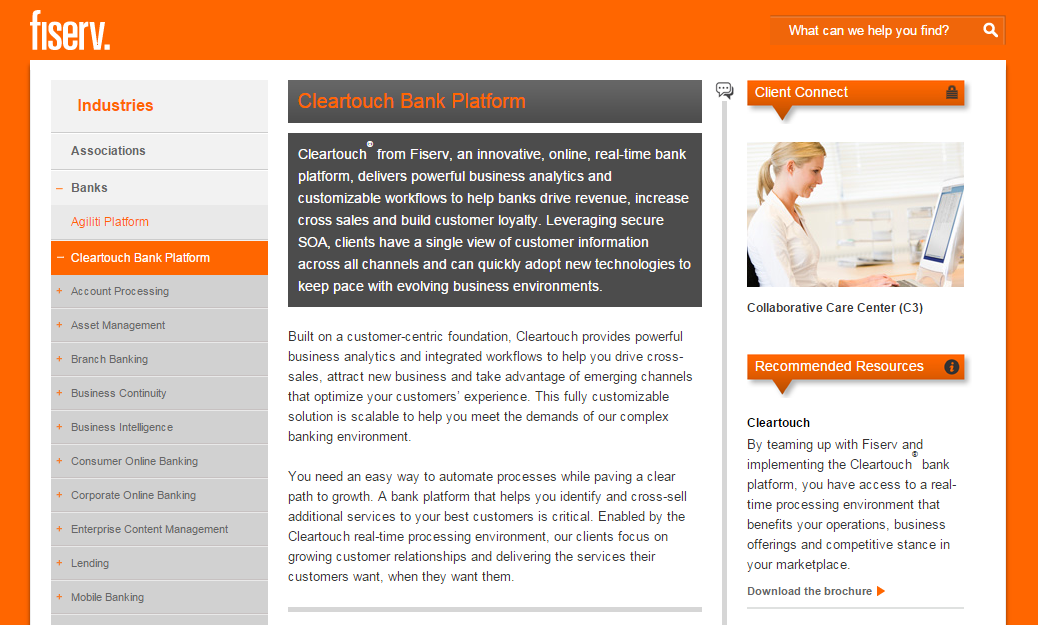This image features a Fiserv bank interface on a white background, framed with an orange trim along the left, right, and top edges. In the upper left corner, the text "Fiserv" is displayed in white. The upper right corner houses a search bar with the prompt "What can we help you find?" displayed in white text next to a magnifying glass icon.

Along the left side of the screen, there is a light gray vertical rectangle labeled "Industries" in orange text, followed by a list of options in black text, including "Associations," "Banks," and the "August Platform" in orange text. Below this is an orange rectangle with the label "ClearTouch Bank Platform" in white text. Further down, there are categories in black text: "Account Processing," "Asset Management," "Branch Banking," "Business Continuity," "Business Intelligence," "Consumer Online Banking," "Corporate Online Banking," "Enterprise Content Management," "Lending," and "Mobile Banking."

The center of the screen features a black rectangle with "ClearTouch Bank Platform" highlighted in orange text. Below it is a larger black rectangle with the following white text: "ClearTouch from Fiserv, an innovative online real-time bank platform, delivers powerful business analytics and customizable workflows to help banks drive revenue, increase cross-sales, and build customer loyalty. Leveraging secure SOA, clients have a single view of customer information across all channels and can quickly adopt new technologies to keep pace with evolving business environments."

Beneath this, on the white background, is additional black text describing the platform: "Built on a Customer Centric Foundation. ClearTouch provides powerful business analytics and integrated workflows to help you drive cross-sales, attract new business, and take advantage of emerging channels to optimize your customers' experience. This fully customizable solution is scalable to help you meet the demands of our complex banking environment. You need an easy way to automate processes while paving a clear path to growth. A bank platform that helps you identify and cross-sell additional services to your best customers is critical. Enabled by the ClearTouch real-time processing environment, our clients focus on growing customer service relationships and delivering the services their customers want and when they want them."

To the right of this text are sections labeled "Client Connect" and "Recommended Resources."